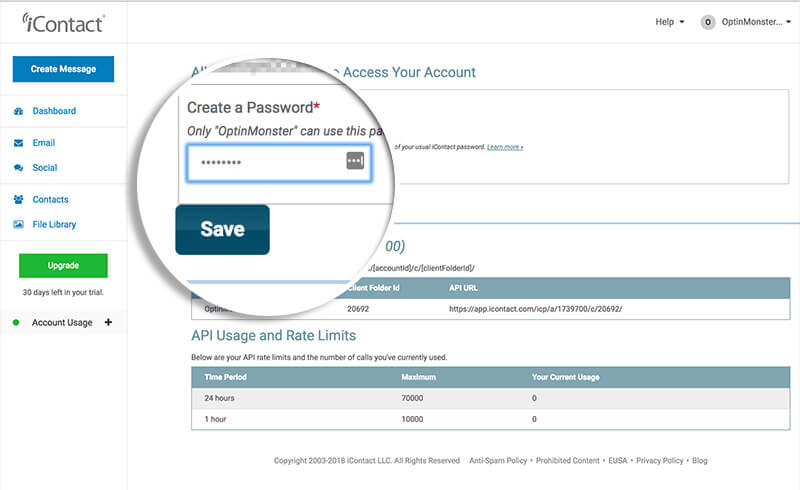This image is a screenshot of a user interface for an application dashboard. At the top left corner, there are several menu options listed: "Eye Contacts," "Create Message," "Redirection Board," "Email," "Social," "Contacts," and "File Library." Just below these options, there is an "Upgrade" button accompanied by the text "30 days left in your trial." 

In the central area, there is a notice regarding "Account Usage," and in the top right corner, there are two dropdown menus labeled "Help" and "Username." Below the "Username" dropdown, there is a "Create a Password" section that contains a magnifying glass icon next to the phrase "Only obtain monster can use this password." 

Further down, you find additional information on "API Usage and Rate Limits." This section includes a table with three columns: "Time Period," "Maximum," and "Your Current Usage." The first row specifies a limit of "70,000" API calls in "24 hours," and the second row details a limit of "10,000" API calls in "1 hour." 

At the very bottom of the image, there is a footer with legal and policy information, including "Copyright 2003 to 2018, Eye Contacts Limited Liability Company, All Rights Reserved, Anti-Spam Policy, Prohibited Contents, EUSA, Privacy Policy," and a link to the "Blog."